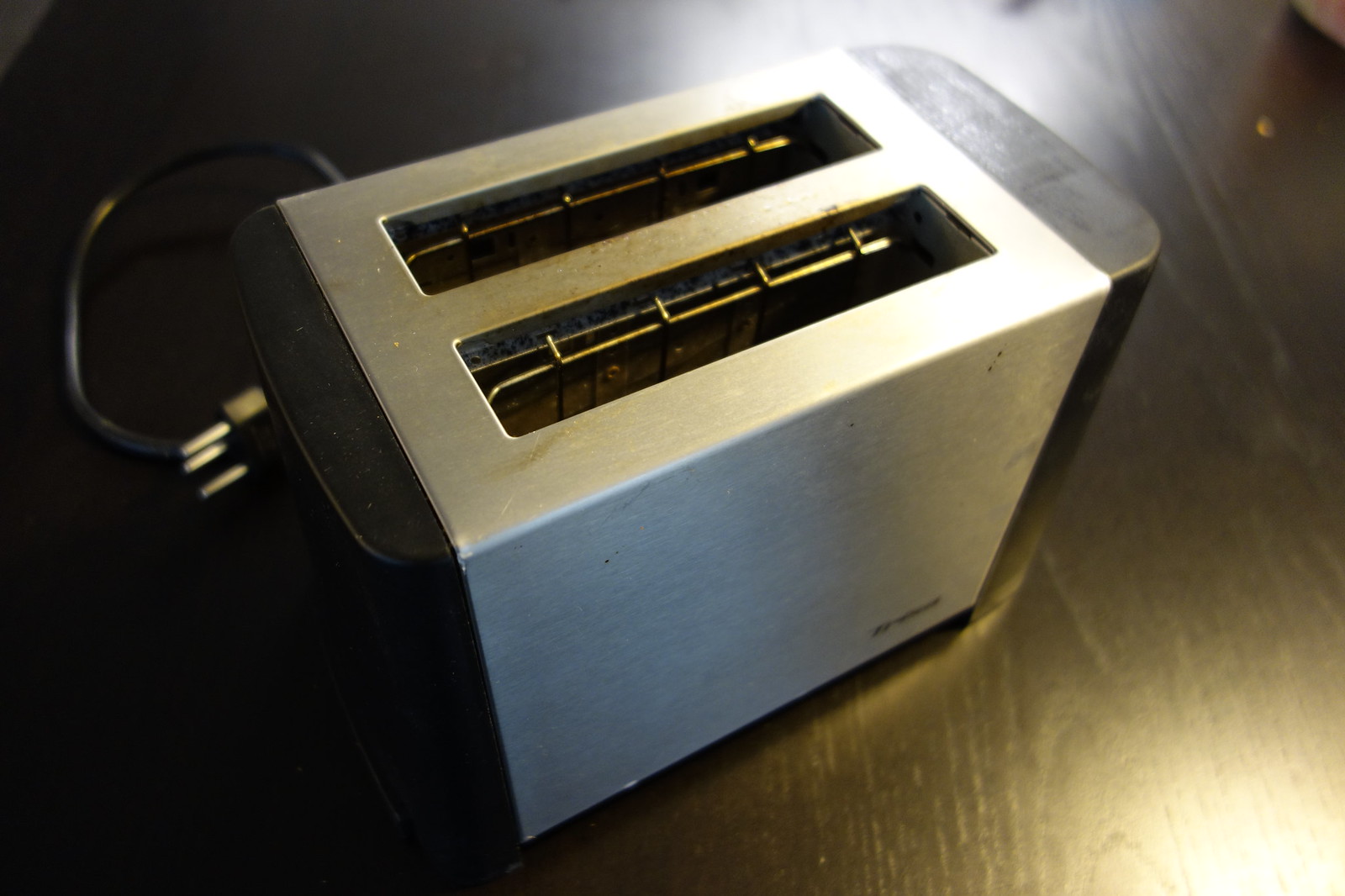This detailed photograph showcases a stainless steel and black toaster in a slightly overhead diagonal view, captured sitting on a dark brown wooden table. The toaster, noted for its rust and grime, is unplugged and its black cord is coiled behind it, with the prongs of the plug visible on the left-hand side. The body of the toaster is predominantly silver, with the narrow ends being black, and features two slots with metal wire grids for holding toast. Although there is branding in black on the bottom right corner, it is too blurry to be decipherable. The image is characterized by reflections of light, showing a yellowish glow in the bottom right corner and a whitish glow in the center top corner, with additional glare spots reflected on the table surface and off the metal top of the toaster. Remnants of crumbs and notable blackened areas inside the slots further illustrate the well-used condition of the appliance.